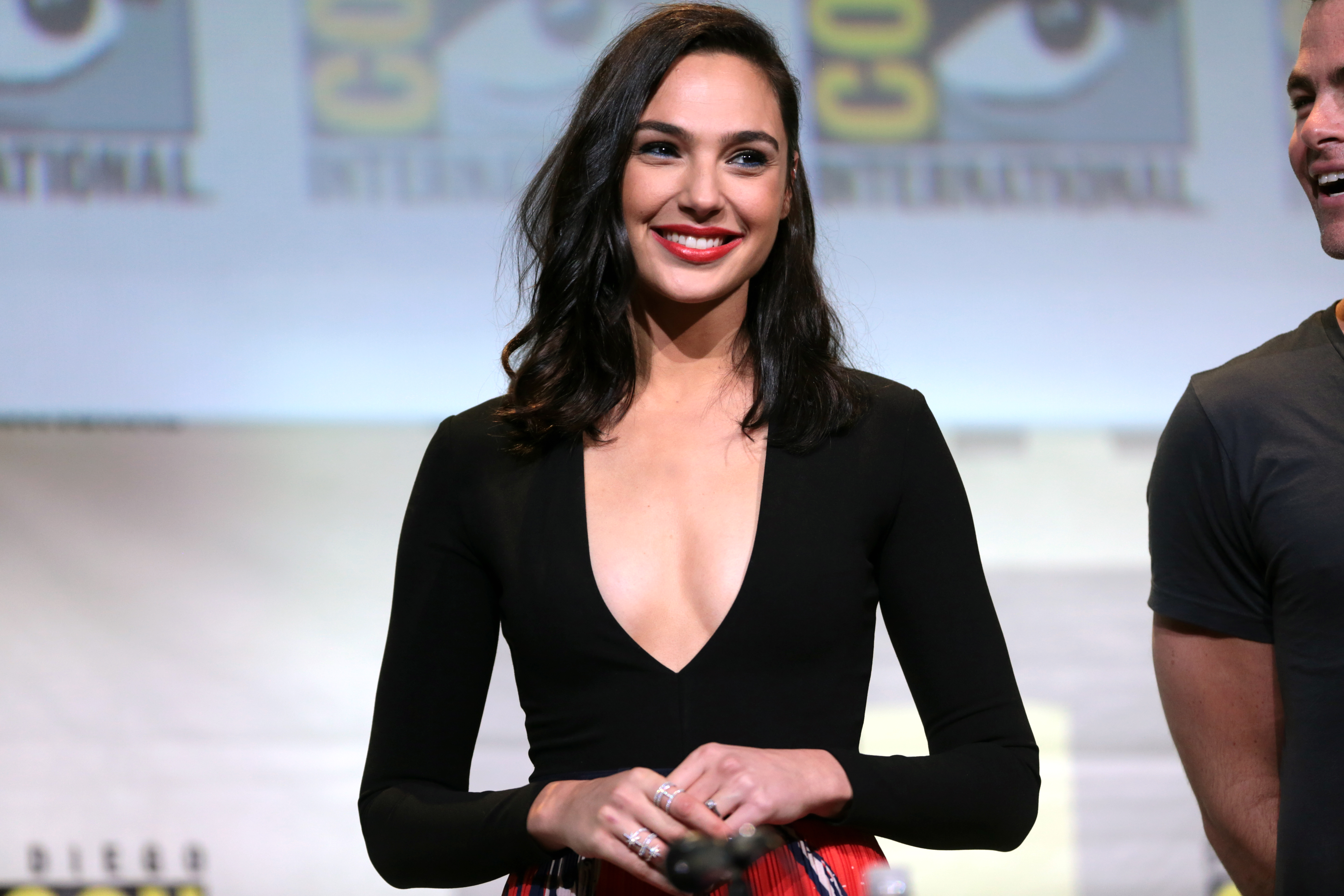The photograph features the famous actress Gal Gadot at Comic-Con, easily recognizable by the repeated Comic-Con logos on the white backdrop behind her. She is standing in the center of the image, facing forward but looking and smiling towards the right with her bright white teeth visible. Her blue eyes are highlighted by black mascara and her dark brown hair, which slightly exceeds shoulder-length, frames her face elegantly. Gal Gadot is wearing a long-sleeved black v-neck top that reveals some cleavage, paired with what appears to be a red skirt, although it is partially obscured. She has a combination of silver rings on her fingers, specifically on her pointer and ring fingers of one hand and her ring finger on the other. She's also sporting striking red lipstick. Next to her, partially cropped out but clearly identifiable, is actor Chris Pine, who is smiling and looking at Gadot. The background is somewhat blurry but distinctly features the Comic-Con logo in yellow letters with an eye design, accompanied by the word "International" written in black letters. The setting is reminiscent of a speaking event, possibly involving a lighthearted moment given Chris Pine's apparent laughter.